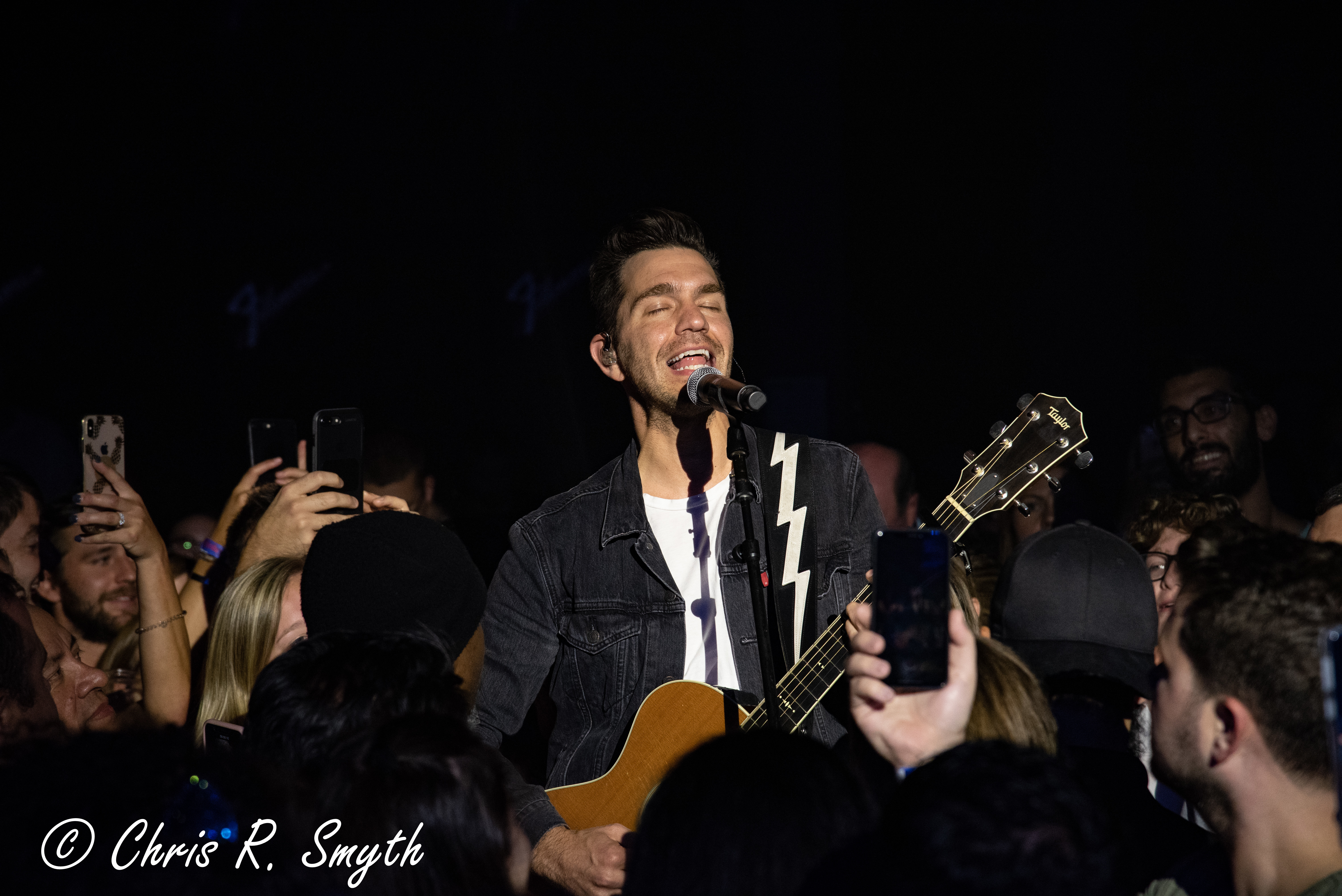The photograph captures an intense moment of a live performance by a musician named Chris R. Smythe, whose name is watermarked in the bottom left corner. The man, positioned centrally in the image, is deeply immersed in his singing with closed eyes and an open mouth, conveying genuine emotion. He grips a guitar, adorned with a strap featuring a white lightning bolt, slung over his left shoulder. Dressed in a white shirt beneath a dark blue jean jacket, Smythe is bathed in focused lighting that highlights him against the dark venue. Surrounding him, a crowd of enthusiastic fans, many with cell phones raised, eagerly capture the performance. The image also details a smiling man in the lower left corner, parts of a blonde woman's hair, the back of a man's head with visible ear in the lower right, and another man's face along the right middle edge, emphasizing the communal and intimate atmosphere of the event.